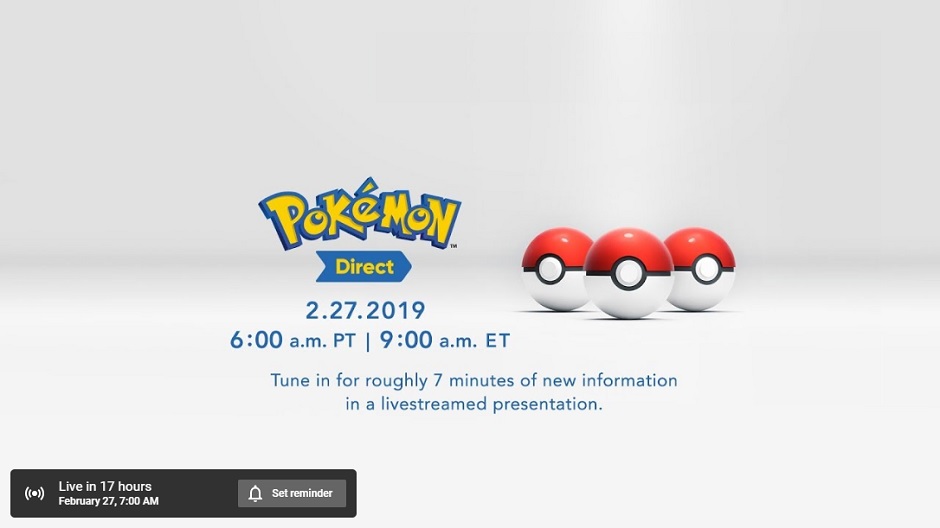The image features a minimalist design with a white background bisected by a faint black line that delineates the wall from the floor, although both surfaces share the same color. 

Positioned slightly to the left of the center, the word "Pokémon" is prominently displayed in bold yellow text, outlined in blue. Directly beneath it, the word "Direct," also in yellow text with a blue background, aligns with the Pokémon logo. Below this, the date "2-27-2019," presented in blue text, specifies times of "6am PT to 9am ET."

At the bottom of the image, a blue text block announces: "Tune in for roughly 7 minutes of new information in a live-streamed presentation." 

In the bottom left corner, a black notification banner reads, "Live in 17 hours, February 27th, 7am," in white text. Adjacent to this notification, a grey button labeled "Set a Reminder" is visible.

To the immediate right of the Pokémon logo, three Poké Balls are perfectly aligned. Each Poké Ball features a red top half, a white bottom half, and a black band encircling the middle, highlighting a central white button.